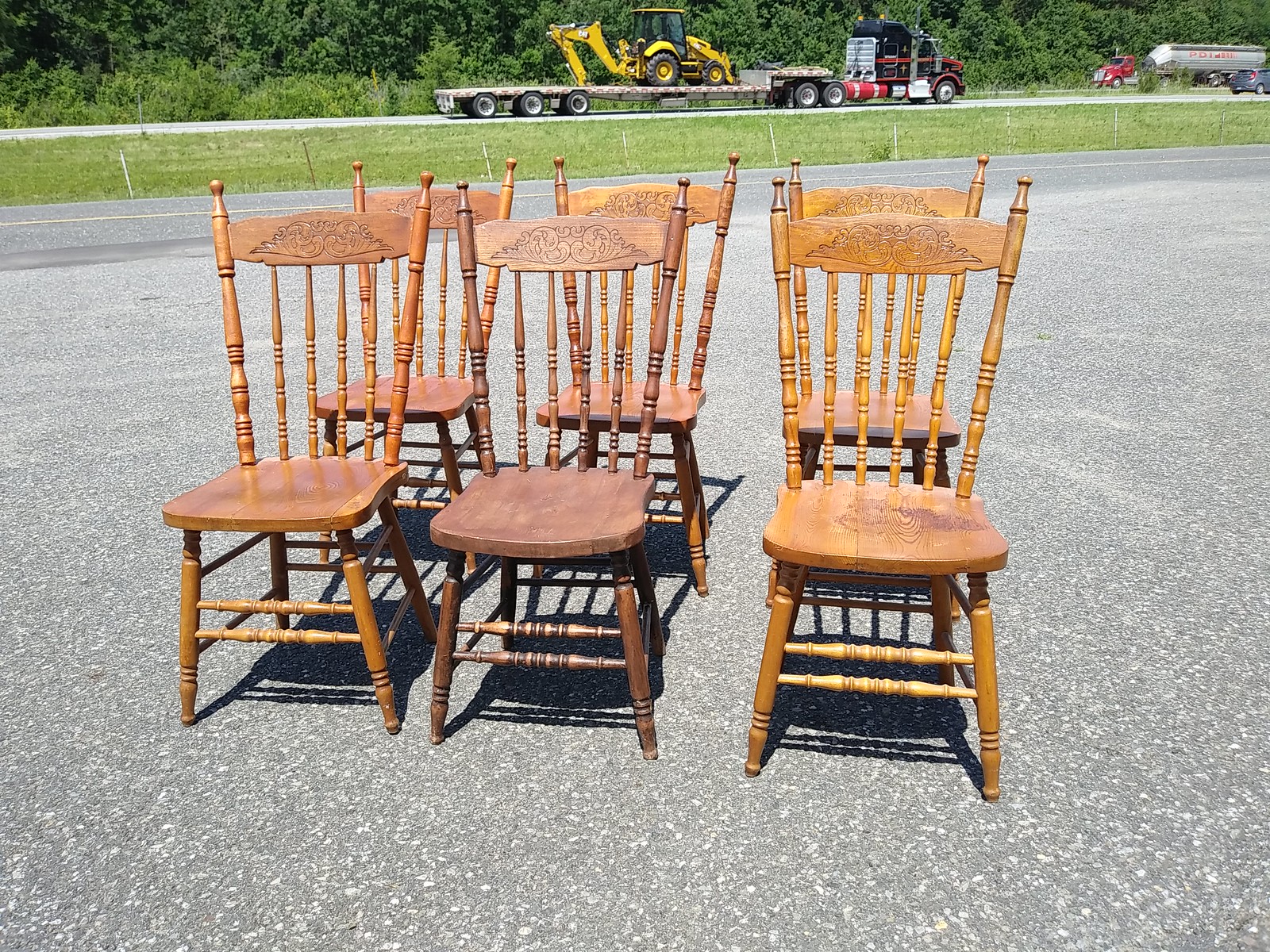This color photograph captures an array of six wooden dining chairs arranged in two rows of three on a textured, light-gray tarmac surface decorated with small white rocks. The chairs, though similar in design, exhibit two distinct styles, differentiated by their shades of brown—some slightly darker than others. Each chair features straight backs adorned with ornamental wooden carvings at the top, and their legs are interconnected by cylindrical wooden poles. The open backs of the chairs showcase a series of decorative vertical wooden poles. The wood appears aged and in need of varnish or stain, with visible cracks hinting at years of use.

In the background of the image, a yellow line marks a road that intersects a green, grassy area. Further beyond, another highway hosts a large truck with a black head and red and grey body. A yellow machine, possibly a tractor, is mounted on a trailer behind the truck. Another smaller vehicle and a grey truck are also visible, suggesting a bustling roadside scene. The farthest reaches of the picture reveal a bushy woodland area under the bright afternoon sunlight, illuminating the entire scene from above. This setting might indicate the chairs are outside a thrift store or a similar establishment for used furniture.